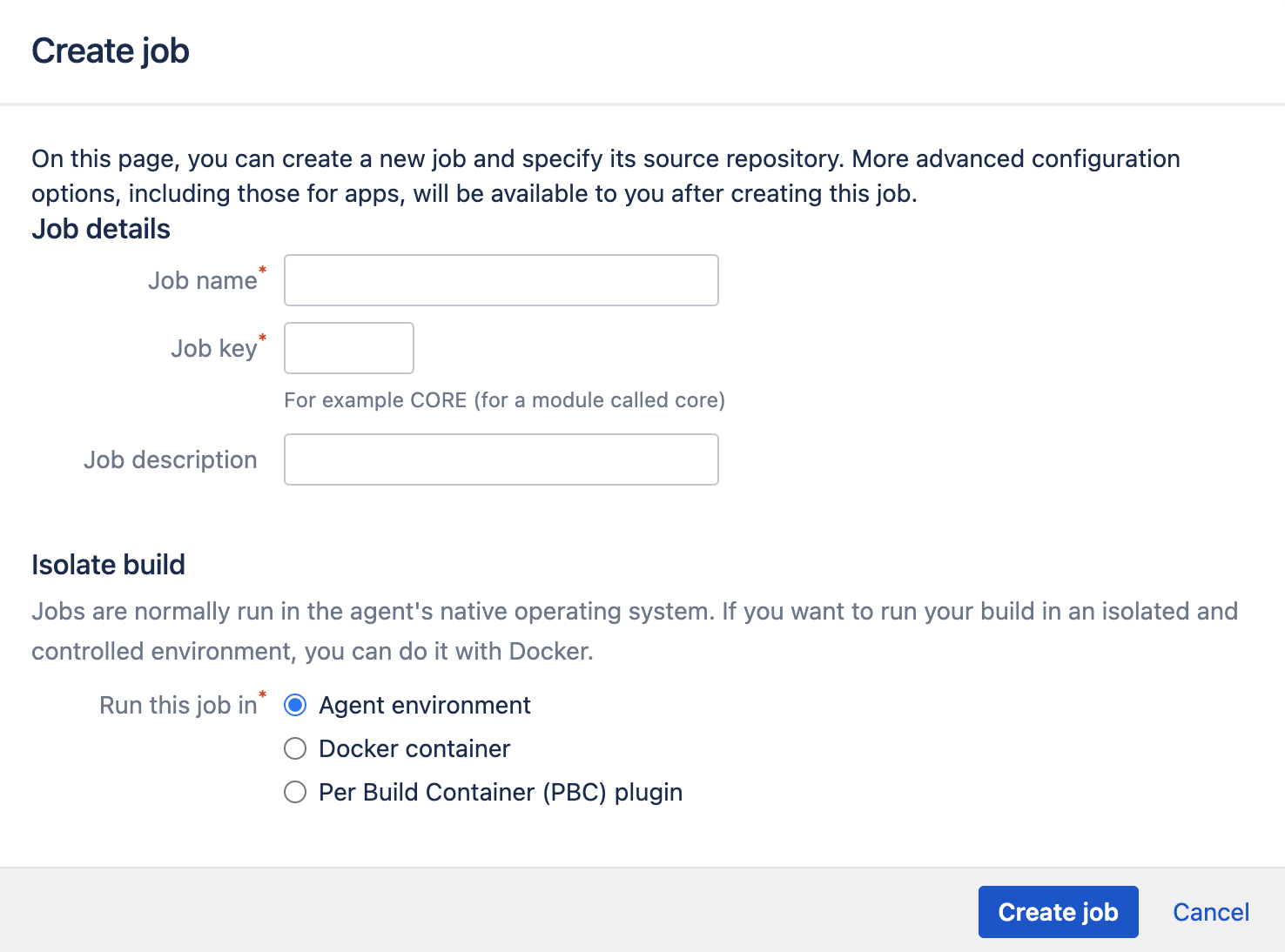This screenshot displays a detailed interface for creating a job within a software application. 

At the top left, the title "Create Job" is prominently displayed in blue font, beneath which a horizontal line delineates the header. Below this line, there is a brief instructional paragraph reading: "On this page, you can create a new job and specify its source repository. More advanced configuration options, including those for apps, will be available to you after creating this job."

Continuing down the page, the section titled "Job Details" contains fields for essential information. The "Job Name" field, marked with a red asterisk to indicate a required entry, is accompanied by a text box for input. Similarly, the "Job Key" field, also marked with a red asterisk, provides space for entering a unique identifier. An example is provided: "For example, CORE (for a module called Core)."

The next section is for "Job Description," featuring a text box for descriptive details about the job.

Below this, another section labeled "Isolate Build" explains: "Jobs are normally run in the agent's native operating system. If you want to run your build in an isolated, controlled environment, you can do it with Docker." The "Run This Job" option, also marked with a red asterisk, presents three choices: "Agent Environment," "Docker Container," and "Per Build Container (PBC) Plugin." The currently selected option is "Agent Environment," indicated by a blue dot.

At the bottom of the window, a gray bar houses two buttons on the right-hand side. The "Create Job" button is white text on a blue background, while the adjacent "Cancel" button is blue text on a white background.